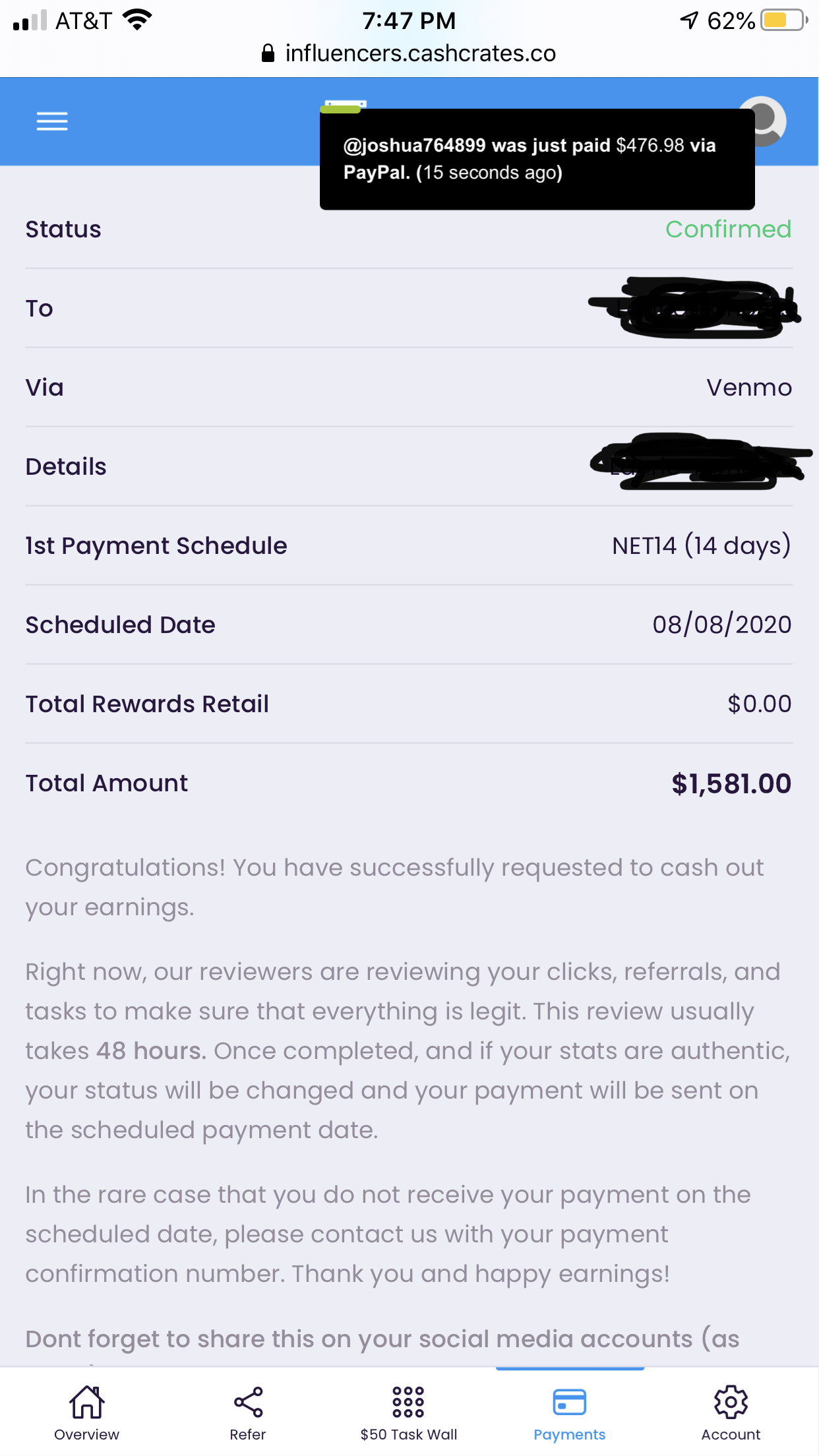The image showcases a smartphone screen displaying a website. The phone in question has a gold color and indicates a battery life of 62%, with an active internet connection through AT&T. The time on the phone is 7:47 p.m. In the top left corner, there's a black lock icon and the URL displayed is influers.cashcrates.co.

The website features a blue navigation bar at the top. Directly below, there is a pop-up notification in a black box stating "Joshua" followed by a payment confirmation notice indicating that Joshua was paid a specific amount via PayPal 15 seconds ago. The status of this transaction is confirmed and marked in green text.

Further down, there is some scratched-out information, indicating some details are obscured for privacy, mentioning payment via Venmo and other specifics. Notably, the first payment is scheduled in "14 days" with a specific schedule date of "08.08.2020". It also lists "Total Rewards Retail" as zero and "Total Amount" as $15,8100.

Within a gray information box, there is a message congratulating the user on successfully requesting to cash out their earnings. It explains that the user's clicks, referrals, and tasks are currently under review to ensure everything is legitimate. This review process typically takes 48 hours, after which, if the stats are authentic, the payment status will be updated and funds will be sent on the scheduled date.
 
The bottom of the screen shows partially cut-off content with navigation icons. The "Payments" icon is highlighted in blue, indicating the current section, with a line above it for emphasis.